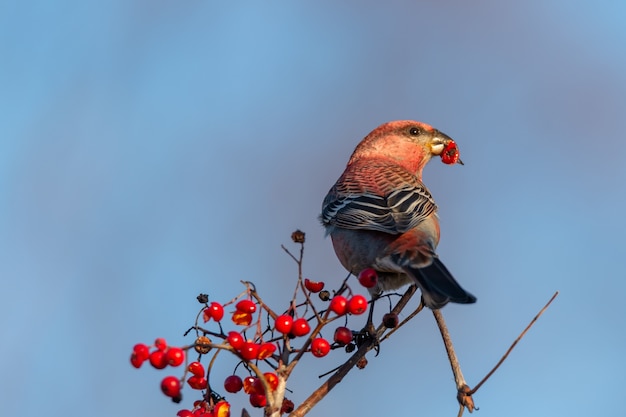This vivid color photograph captures a small, multi-colored bird perched on a thin branch of a cherry tree. The bird, facing away but slightly turned to the right, displays its striking plumage detailed with an array of vibrant hues. Its head is a brilliant red with a small black eye and a black and white beak, from which it holds a red berry. The back and wings feature an intricate pattern of black and red feathers with distinctive black and white stripes outlining the edges. The neck exhibits similar black and white colors, extending to a blue bottom with additional red feathering in between.

The bird's black tail feathers add contrast to its more colorful upper body. Surrounding the bird, the bare branches of the cherry tree are adorned with clusters of bright red berries, some ripe and round, others in stages of decay, creating a dynamic and natural setting. This picturesque scene is set against a backdrop of a serene, cloudless sky that transitions from light blue to a soft purple near the center, enhancing the overall vividness and tranquility of the image.